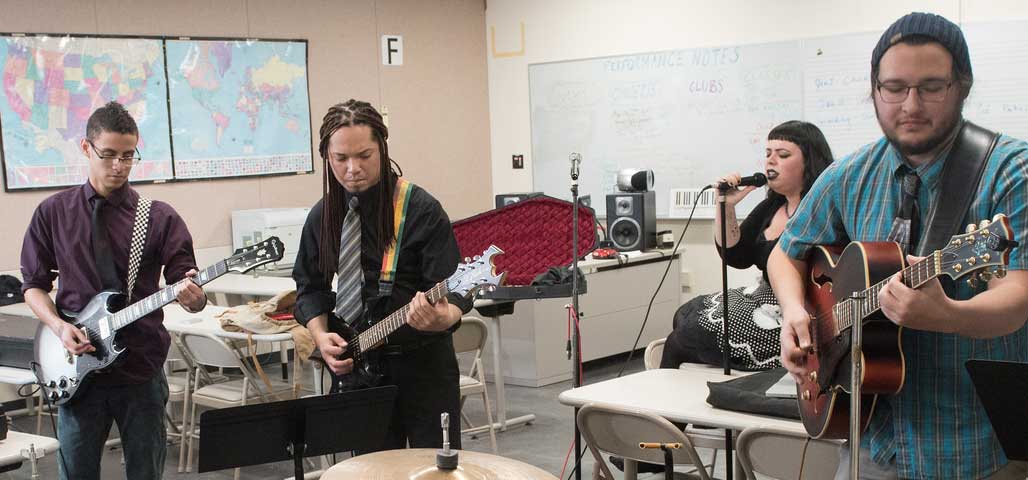This image captures a band of four people, three guys and one girl, performing music in a classroom setting. The room has the typical academic décor, featuring desks, chairs, maps of the United States and the world, a whiteboard, speakers, and a drum set partially visible through a cymbal. The classroom walls are painted a muted beige and darker brown tone, and there's a large "F" prominently displayed on one wall, indicating it might be Classroom F.

The two guys on the left are playing electric guitars. The one furthest left is wearing glasses, a purple shirt, a black tie, and jeans. The next person, who also has a tie, is dressed entirely in black and has dreadlocks. The guy on the right is playing an acoustic guitar and wears a blue beanie and a turquoise shirt. The centerpiece of the group is the girl, singing into a microphone. Although partially obscured by the guy on the right, she stands out with her black outfit, black hair, and black lipstick. Despite their focused expressions, with the girl having her eyes closed, there are no other students visible, adding a sense of intimacy to their jam session.